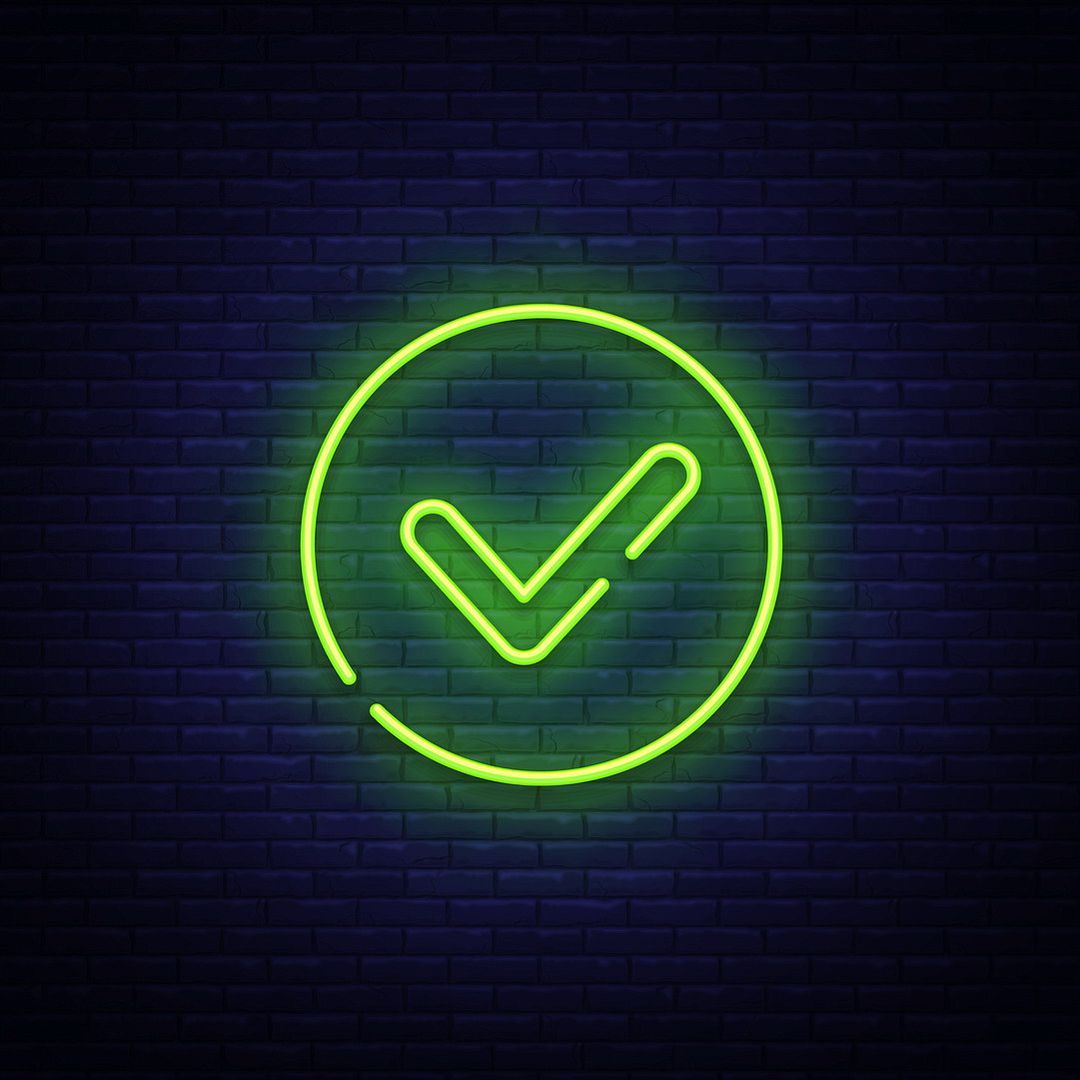This close-up photo features a striking neon sign mounted on a blue brick wall. The wall, dark along the perimeter and gradually lighter towards the center, is illuminated by the green neon light. The neon sign comprises a nearly complete circle with a small break at around the seven o'clock position, encasing a partially connected check mark. The check mark starts from the right and extends leftward, with a similar break in continuity. Both elements, outlined in bright green neon, cast a subtle reflection on the surrounding bricks, which exhibit hues of dark blue and purple. The intensity of the light creates a bright focal point against the otherwise shadowy backdrop, suggesting a modern and possibly trendy setting, like an office, bar, or startup company.